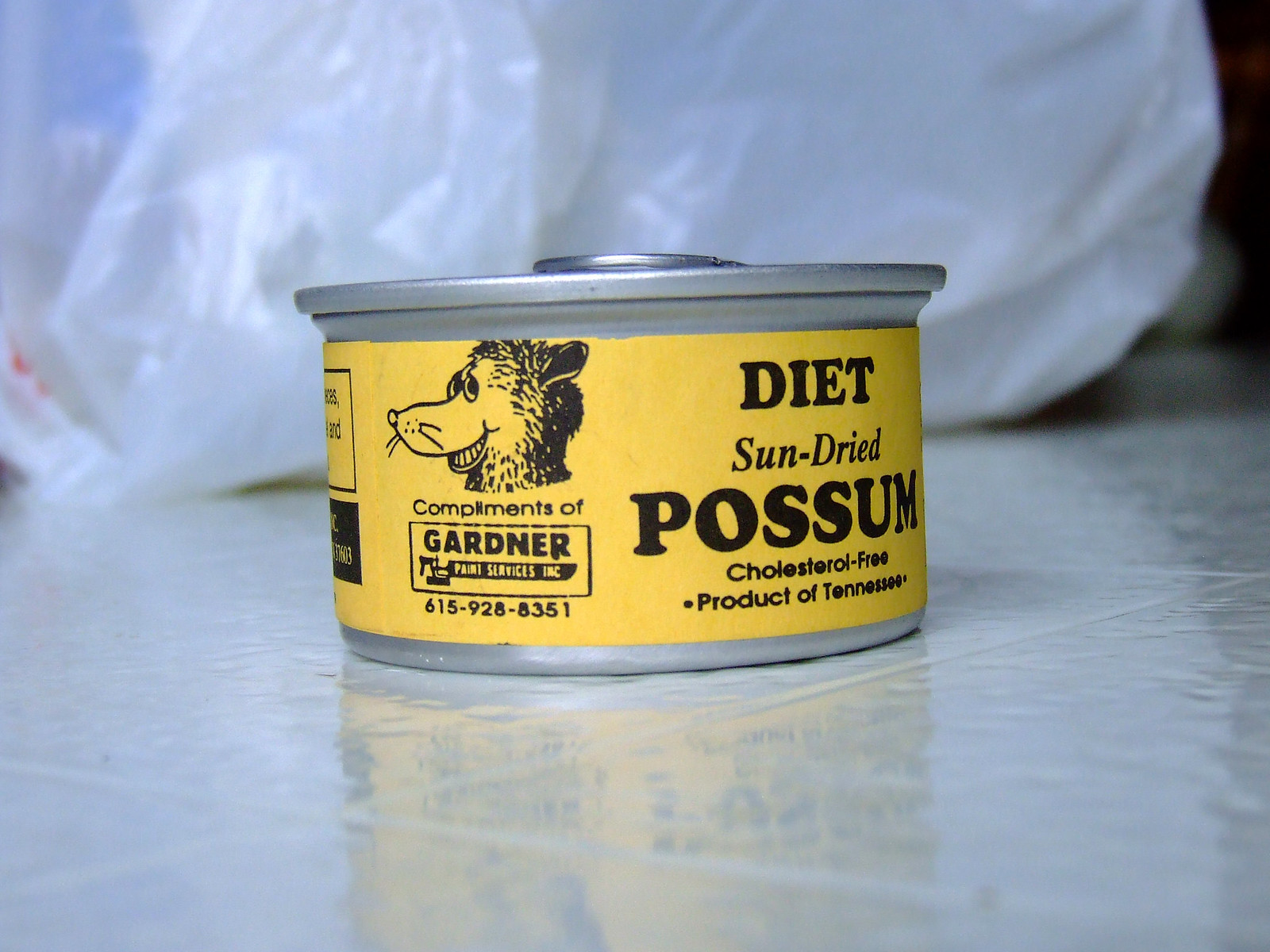The image features a close-up of a small, prepackaged aluminum can of food, prominently displayed on a shiny white ceramic countertop. The can is circular and positioned at a slight angle, showcasing a light golden yellow label that wraps around it. The label includes a prominent drawing of a smiling possum facing left, under which the text reads "compliments of Gardner Print Services Incorporated" along with a phone number, 615-928-8351. The primary text on the can, written in black, declares it as "diet sun-dried possum," indicating it is cholesterol-free and a "product of Tennessee." The top of the can features a pull-tab for easy opening. The background includes a blurred plastic or cellophane bag and slight shadowing in the right corner, enhancing the focus on the can itself.